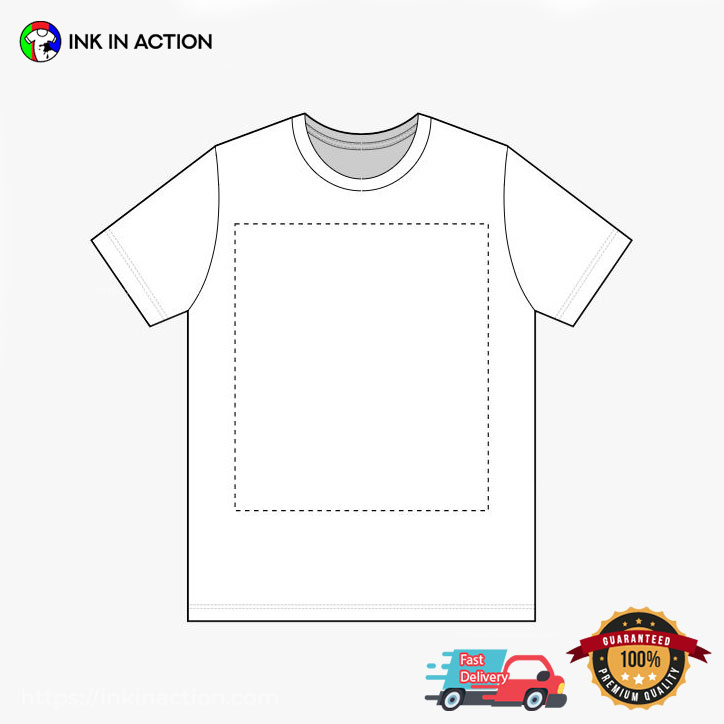The image displays a clean, light gray background with a simple white t-shirt illustration at its center. The t-shirt is depicted with short sleeves, a rounded neck, and a prominent dotted line forming a large rectangular area on the front, indicating a printable zone. In the upper left corner, the text "Ink in Action" is presented in bold black letters beside a small circle containing colorful splotches of green, red, and blue. Within this circle, another white t-shirt appears against the multicolored background. In the lower right corner, there is a gold and black badge that reads "Guaranteed 100% Premium Quality," adorned with a red banner. Adjacent to this badge, a red truck with a blue cargo area is illustrated, bearing the words "Fast Delivery." The overall design suggests an advertisement or web interface for a custom t-shirt printing service, emphasizing quality and prompt delivery.